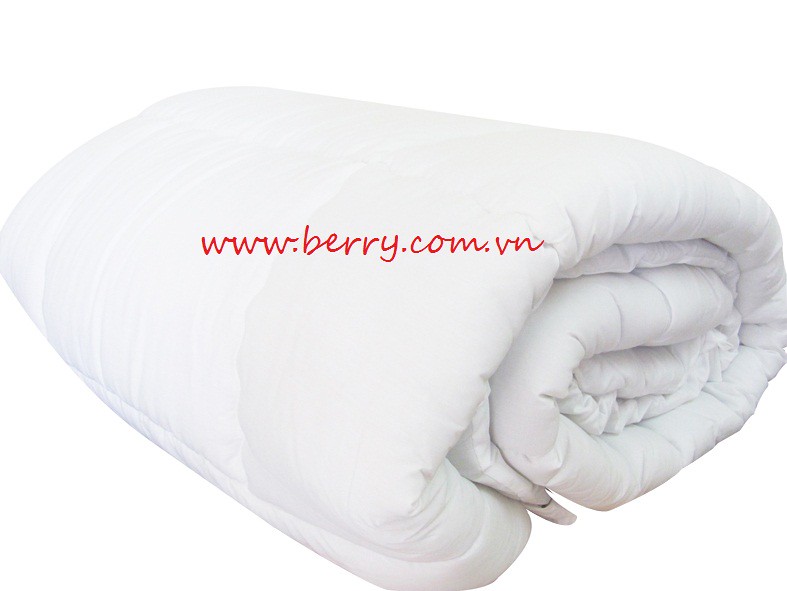The image features a large, white blanket, rolled up in a manner similar to a sleeping bag or a jelly roll, showcasing a thick and fluffy texture. The blanket, possibly a feather or down duvet, is distinguished by its square box stitching pattern and is wrapped several times, allowing viewers to see both the side and one end. It stands out against a white background due to its slightly brighter white shade. Prominently displayed across the center of the image in red, handwritten-style text is the website "www.berry.com.vn," indicating where the product can be purchased. The overall simplicity of the image, with its clean, borderless background, suggests it might be a promotional photo typically used on an online web store or shop.